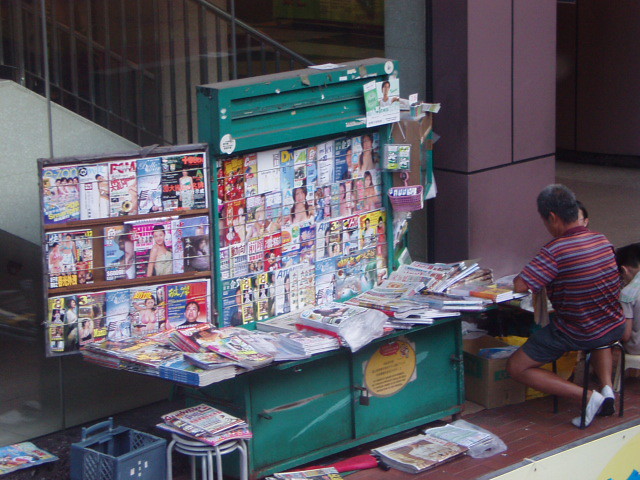The color photograph depicts a vibrant setting centered around a dark greenish-blue magazine stand crafted from wood, characterized by a base with two drawers and an upright portion for display. The stand is cluttered with various magazines, both displayed in overlapping rows and stacked untidily on the counter. Situated on the right-hand side of the image, a man with short dark hair, dressed in a red and blue striped t-shirt, blue shorts, and white shoes, sits on a stool. His back is turned to the camera, with his figure occupying the bottom right corner of the frame. To the left of the stand, additional storage bins and another stool are visible, each also holding magazines. In the background, above the man, a divided red pillar is seen alongside a glass pane. The setting suggests a public space, possibly a mall or the exterior of a popular building, with stairs that reinforce the bustling, communal atmosphere. The floor beneath the scene is a notable red, further adding to the colorful composition of the photograph.